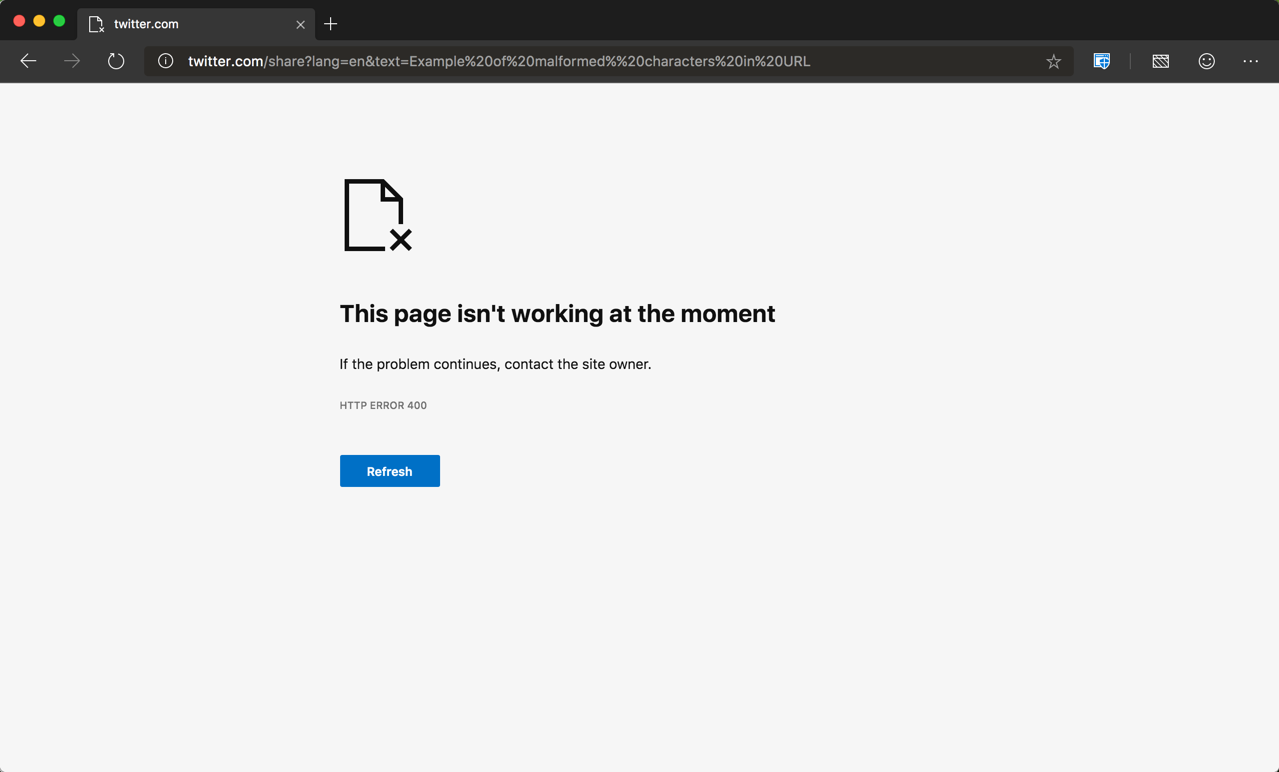A screenshot of a web browser displaying a Twitter.com error page. At the top, a black search bar is visible along with the Twitter logo. The main content of the page features a large 'X' and a message indicating that the page is not working at the moment. It suggests that if the issue persists, the user should contact the site owner. The page also shows an HTTP error code 400 and a refresh instruction. This error message is repeated multiple times, emphasizing the temporary unavailability of the Twitter page.